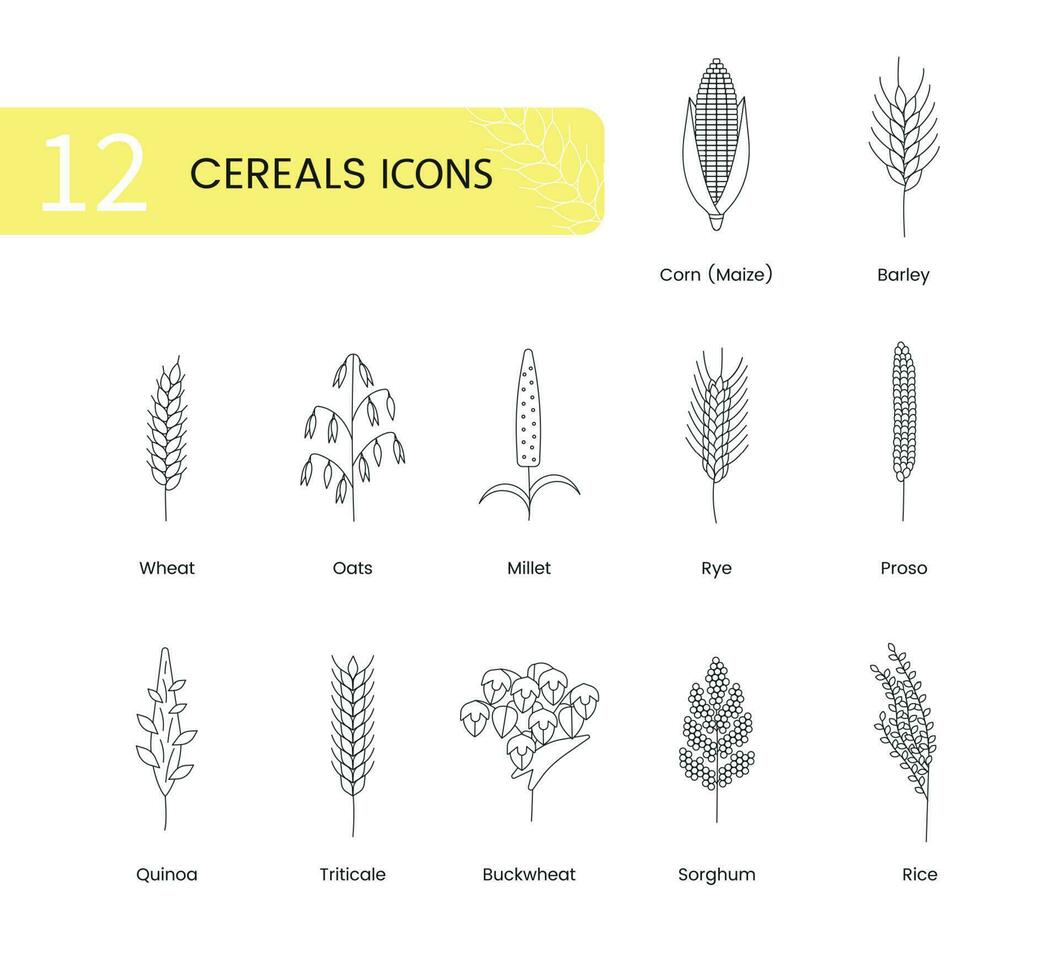This image features a detailed chart of cereals, displayed on an all-white background. In the upper left corner, a yellow banner highlights the title "12 Cereals Icons." The number 12 is prominently displayed in white, accompanied by black text and a white outline of a grain symbol. Below the title, the chart showcases twelve hand-drawn, black-and-white illustrations of various cereal grains, each labeled clearly.

Starting from the top left, the first illustration depicts corn (maize), presented as a vertical plant with a classic corn cob. Next to it is barley, represented by a wheat-shaped plant, followed by wheat, another grain-shaped plant illustration. Oats are uniquely detailed with hanging seeds dangling from each leaf, making it stand out among the illustrations. Millet is depicted almost like a popsicle, with seeds clustering in the middle. Rye, proso, and quinoa follow, each illustrated as distinct grain-like plants, with quinoa also resembling a popsicle but with leaves extending from its sides. Triticale, another wheat-shaped plant, sits next to buckwheat, which is portrayed with strange, acorn-like ends. Sorghum is depicted with circular seeds, and finally, rice is shown as a typical grain-shaped plant, concluding the sequence. All illustrations are rendered in a simple yet clear black-and-white style.